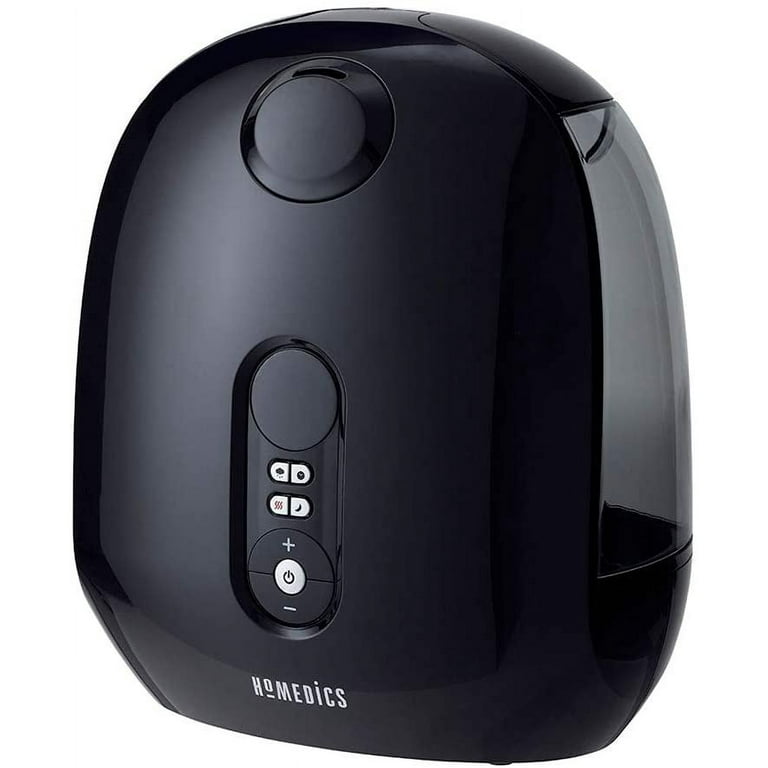The photograph showcases a sleek, black electronic device resembling a high-end humidifier, positioned slightly tilted to the left. The device features an oblong, pod-shaped design with a flat bottom and a curved top. Prominently displayed in white letters at the bottom center of the front panel is the brand name, "Homedics."

At the very top, there's a large, circular button with a vent hole, indicating where the mist may come out. Below it, another black circle contains a display. The control panel, centered on the front, includes four silver buttons with icons depicting different functionalities: a crescent moon, swirly lines for heat, a cloud with rain, and a circle. Directly below this set of buttons is a circular control with a power button at the center, flanked by a '+' on top and a '-' on the bottom.

The right side of the device features a transparent water tank, likely used for storing water to produce mist. The entire image is captured in portrait orientation, with the angle allowing a clear view of both the front control panel and the water tank.